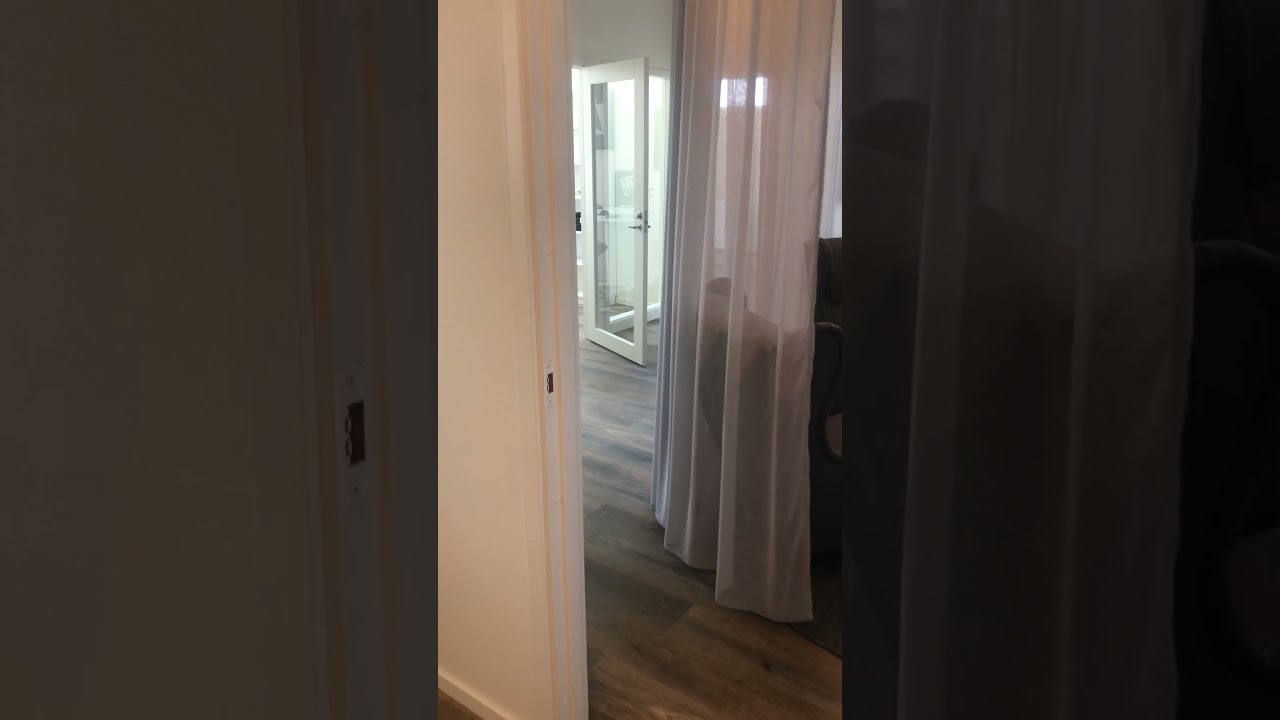The detailed photo depicts an interior view from a camera situated in a hallway of a home. The composition centers on an open doorway framed against an off-white wall on the left and sheer white curtains on the right, both in shadow. The flooring is a dark brown hardwood that stretches across the image, providing a warm contrast to the pale walls. Through the doorway, an open glass door is visible, adorned with a handle and slightly ajar, allowing a glimpse of a dimly lit space beyond, possibly a living room. The ambiance outside the glass door appears to be gray, contributing to the subdued lighting that casts the room in shadow. This scene seems to be part of a larger triptych, as it is flanked by black panels on either side. No text or people are present in the image, creating a quiet, contemplative mood.